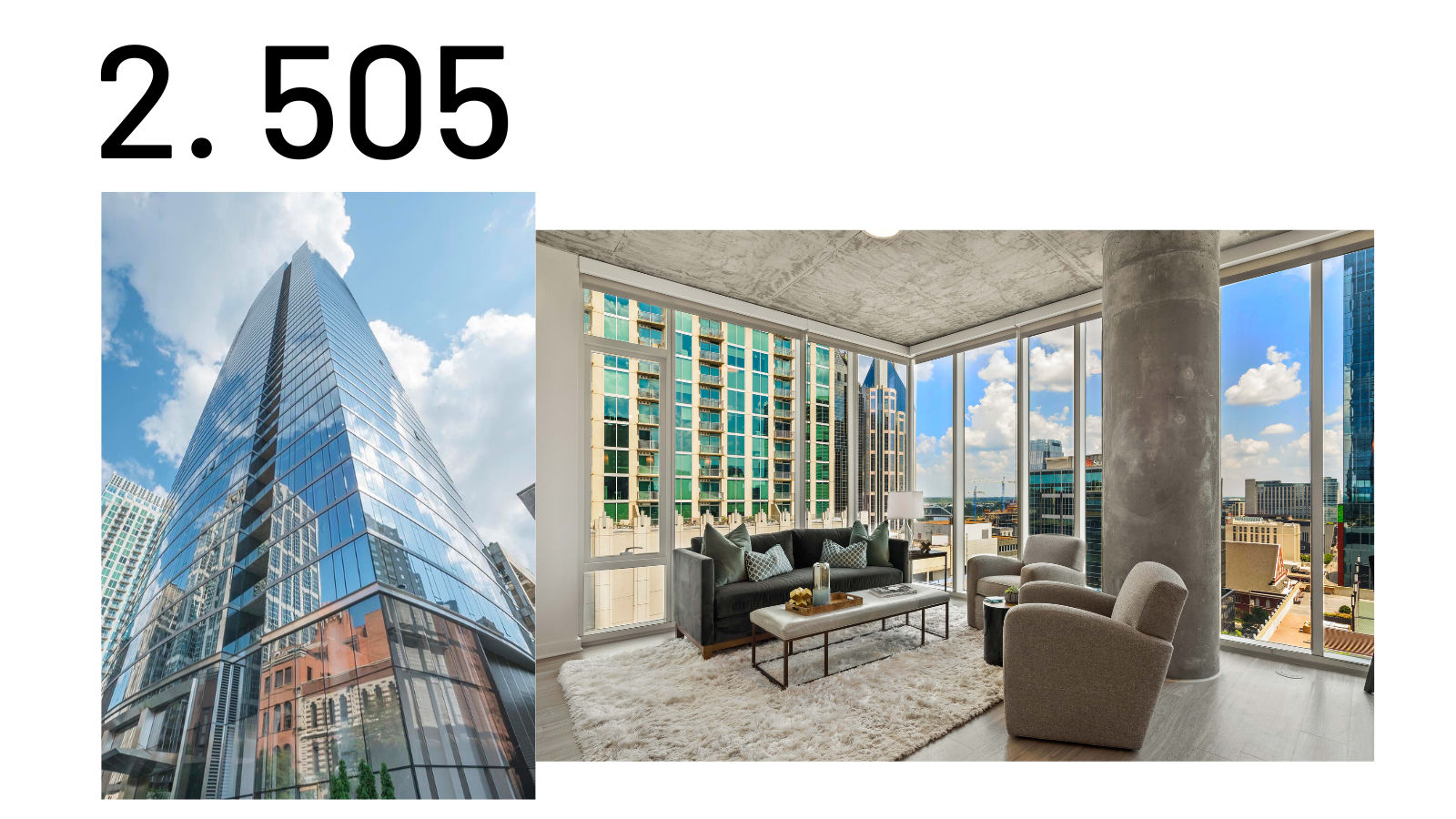The website prominently features the large number "2.505" displayed at the top in strikingly large font. Below this number, there is an impressive photograph of a skyscraper. The picture is taken from the ground level, emphasizing the grandeur of the building as it soars into the sky. The skyscraper's mirrored facade captures and reflects the surrounding environment, including the blue sky dotted with clouds and neighboring buildings, creating a visually captivating scene.

Adjacent to this vertical image of the skyscraper is a horizontal photograph that offers a glimpse into an elegant living room. The space is characterized by its openness and abundance of natural light, as the walls are made entirely of floor-to-ceiling windows without curtains. The room is tastefully furnished with a tan area rug, a gray couch, and a matching tan coffee table flanked by two tan chairs. Dominating the space is a large pillar, seemingly wrapped in soft material akin to carpet. Through the expansive windows, one can see an adjacent building on one side and a panoramic view of the city's skyline, complete with distant buildings, the sky, and clouds, on the other. The room also features hardwood floors, adding to its luxurious ambiance.